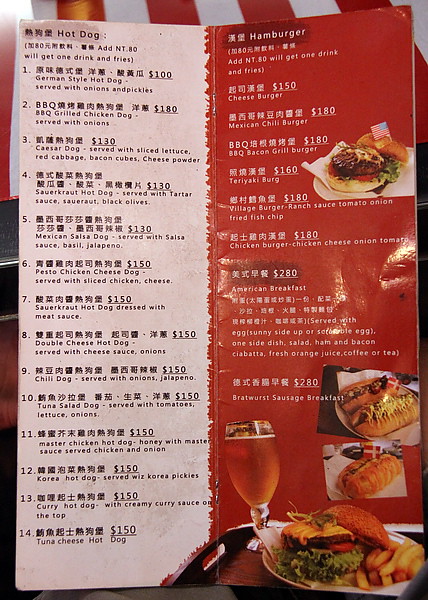This image showcases a well-designed menu, featuring a combination of Asian script and English text, making it accessible to a diverse audience. The menu unfolds like a brochure with a pleasing contrast of light tan on one side and vibrant red on the other, set against a backdrop of red and white stripes. 

On the light tan page, the topmost item listed is "Hot Dog," while the red page starts with "Hamburger." The light tan side is meticulously numbered from 1 to 14, with each entry presented first in Asian script followed by its English translation. The delectable offerings on this side include options such as a German-style hot dog, BBQ grilled chicken dog, Caesar dog, sauerkraut hot dog, Mexican salsa dog, and a pesto chicken cheese dog.

The red side of the menu showcases a variety of burgers. The listings start with a classic hamburger and cheeseburger, followed by enticing variations like a Mexican chili burger, BBQ bacon grilled burger, and a teriyaki burger, among others.

In the bottom right corner of the red page, there is an inviting image of a delicious-looking burger served on a plate alongside a clear, stemmed glass filled with refreshing beer. This visual aids in enticing the customers, complementing the mouth-watering descriptions of the menu items.